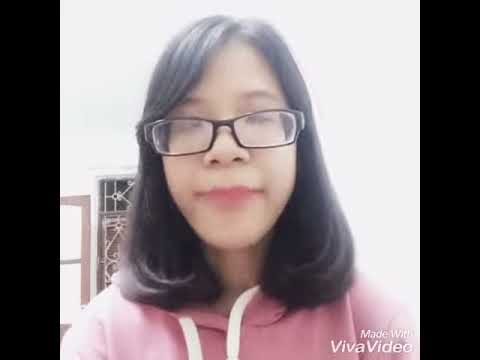The photo is a close-up image of a young Asian woman with shoulder-length, slightly curled-under, black hair. She is wearing black-rimmed glasses, which are tipped slightly forward towards the tip of her nose. She is dressed in a pink hoodie with white laces. Her eyes are closed, and her mouth is shut, giving her a neutral expression. The background features a white wall, a window with white grill work that may be part of a door, and another window or door frame with glass to the left. The photo, well-lit with a white backdrop, includes text in the bottom right-hand corner that reads "Viva Video." This suggests that the image may have been captured during a video chat or recording using the Viva Video app.